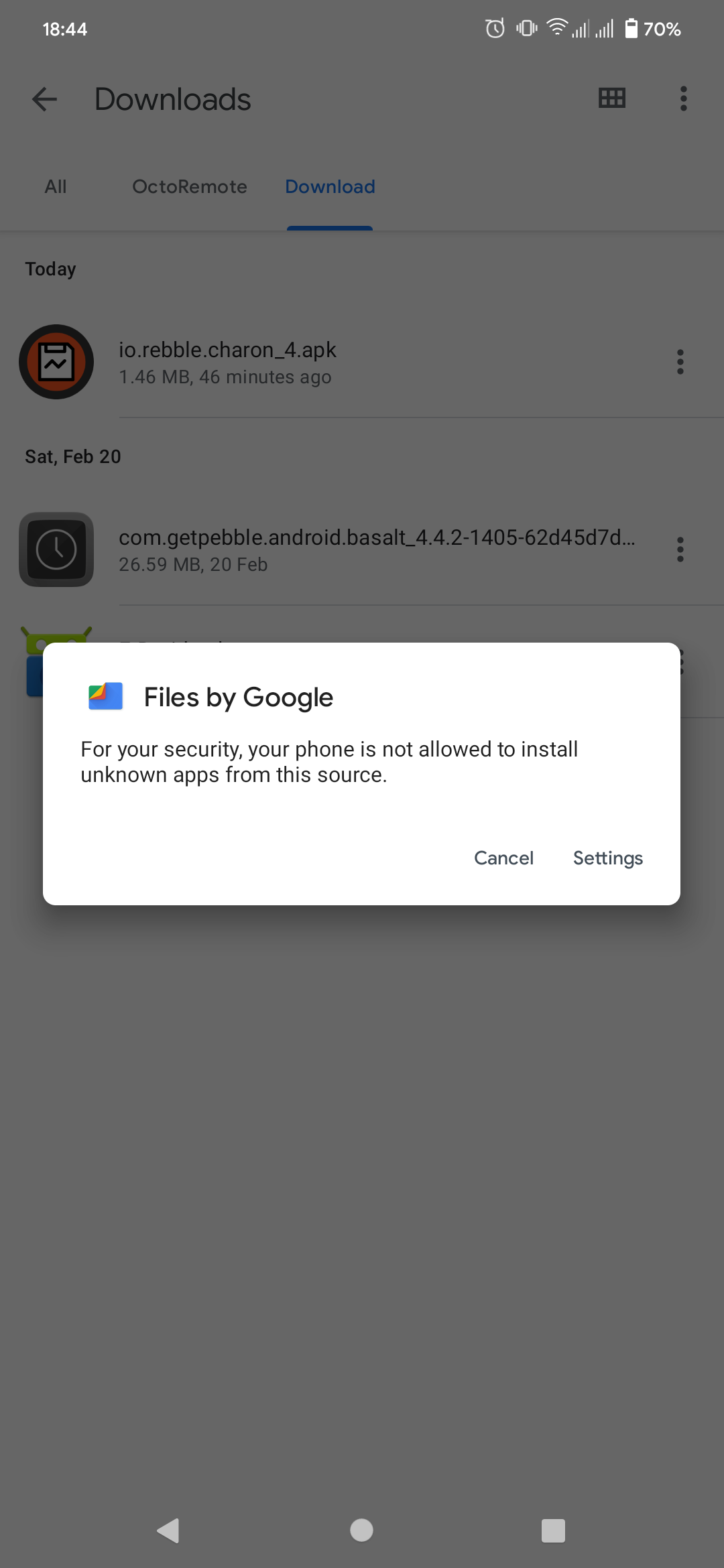In the image, a mobile device, identified as an Android, displays several screenshots. In the top left corner, the device's time is shown as 18:44, indicating it is 6:44 PM. On the top right, various status icons are visible: an active alarm icon, vibration mode icon, Wi-Fi connection icon, and two network signal bars. SIM 1 indicates 4 out of 5 bars, while SIM 2 shows full signal strength with 5 out of 5 bars. Additionally, the battery is at 70% capacity.

The screen is presenting a list of downloads. The sections displayed include:

- "Downloads" tab with sub-categories like "All" and specific files.
- A file named "octoremote" identified as "io.rebi.sharon.4.apk," which is 1.46 MB in size and was downloaded 6 minutes ago.
- Another file named "com.getpebble.android.baseout," with the version "4.4.2-1405-62d45d7d," sized at 26.59 MB, downloaded on the 20th of February.